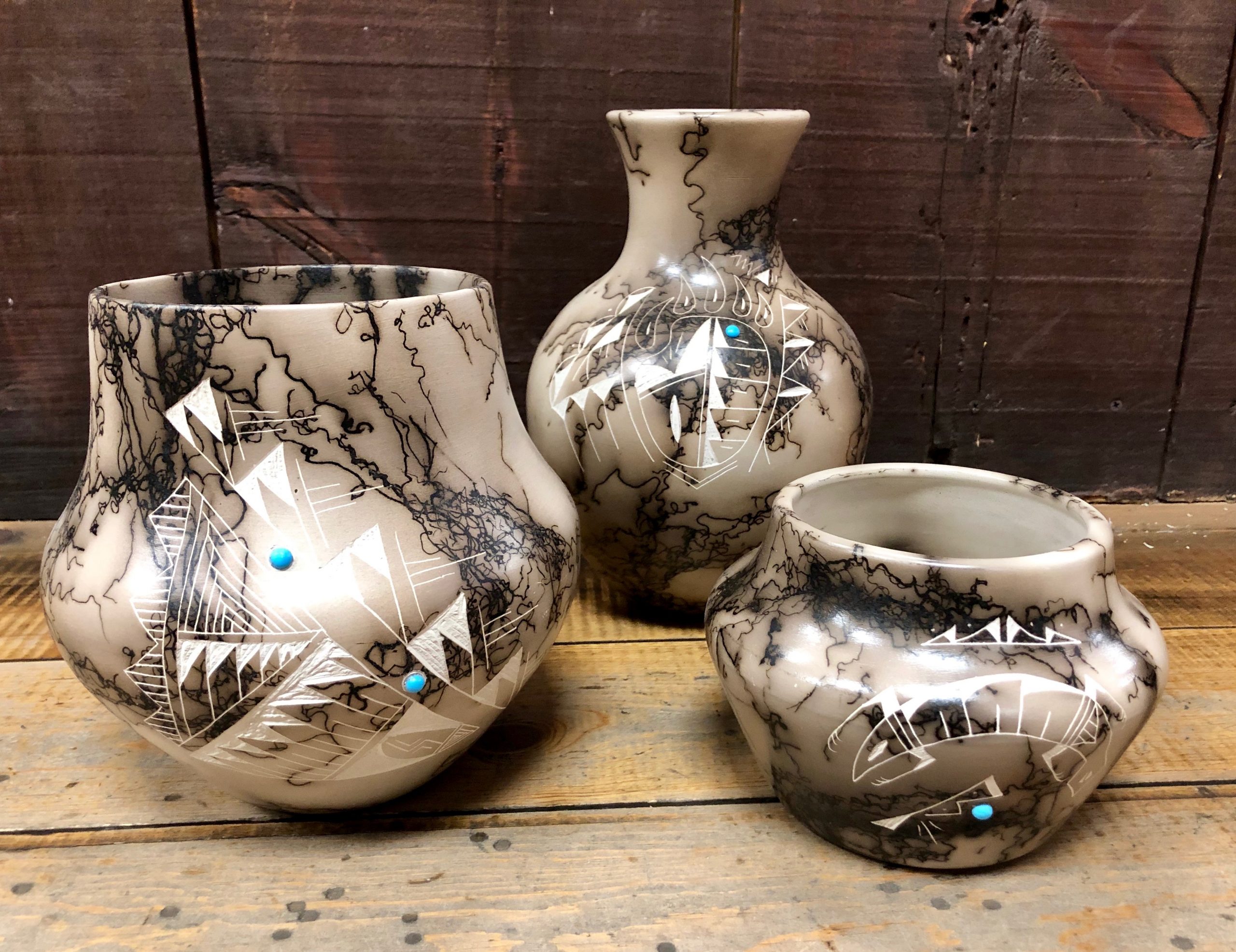This horizontally oriented photograph features a captivating collection of three artfully decorated ceramic vases displayed on aged, distressed hardwood flooring with a darker wooden backdrop showing visible knots. The ceramics are predominantly white and ivory with grayish tones, accented by striking black marbling streaks and decorated with delicate, ancient native-esque linear patterns.

The vase on the left is the largest, resembling a pot belly shape that tapers into a wide bowl opening. It features prominent dark marbling patterns and a turquoise blue dot among the intricate white designs. The center vase is taller with a bulbous base that narrows into a neck, flaring out again at the top. It is similarly adorned with black marbling and a striking turquoise dot, complemented by white triangular and linear motifs. The third vase on the right is more squat and stout, with a large, rounded beveled lip and a narrower circumference. It too carries the signature black and white marbling and an accent turquoise dot.

Each piece, while unique in shape and size, shares a coherent artistic theme that ties the collection together, making it an intriguing addition to any ceramic art collection.